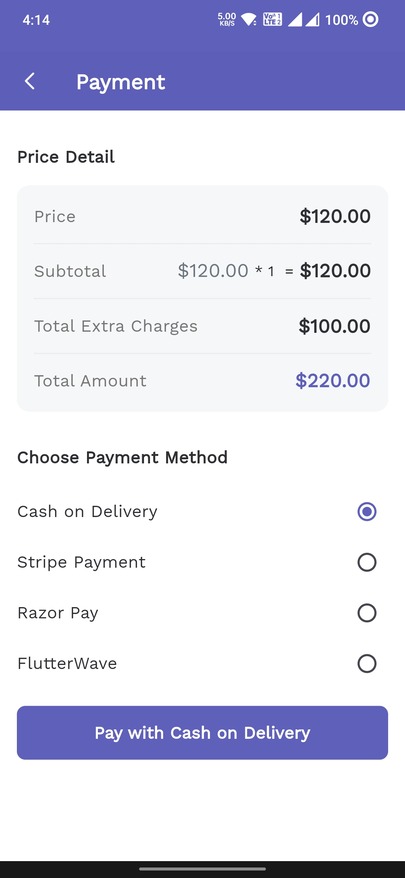At the top of the page, a blue square displays the number "414." Adjacent to this are emblems that represent user-specific details and charge information, indicating "100%." Below this section, an arrow points to the left and the word "Payment" is written in white letters. Underneath, the words "Price Detail" appear in black letters.

Next, a gray box contains the following details:
- "Price: $120"
- "Subtotal: $120 * 1 = $120" (with an asterisk denoting a footnote or special mention)
- "Total Extra Charges: $100"
- "Total Amount: $220"

The amount "$220" is highlighted in red ink, while other amounts are written in dark black. The terms "Price," "Subtotal," "Total Extra Charges," and "Total Amount" are in light gray.

The section labeled "Choose Payment Method" is displayed in bold black text. Below, there are several options:
- "Cash on Delivery" with a blue filled circle indicating selection
- "Stripe Payment" with an empty, black-outlined circle
- "Raise Your Pay" with another empty circle
- "Flutterwave," also with an empty circle

At the bottom, a blue rectangle with white letters states "Pay with Cash on Delivery," and underneath lies a small black rectangle.